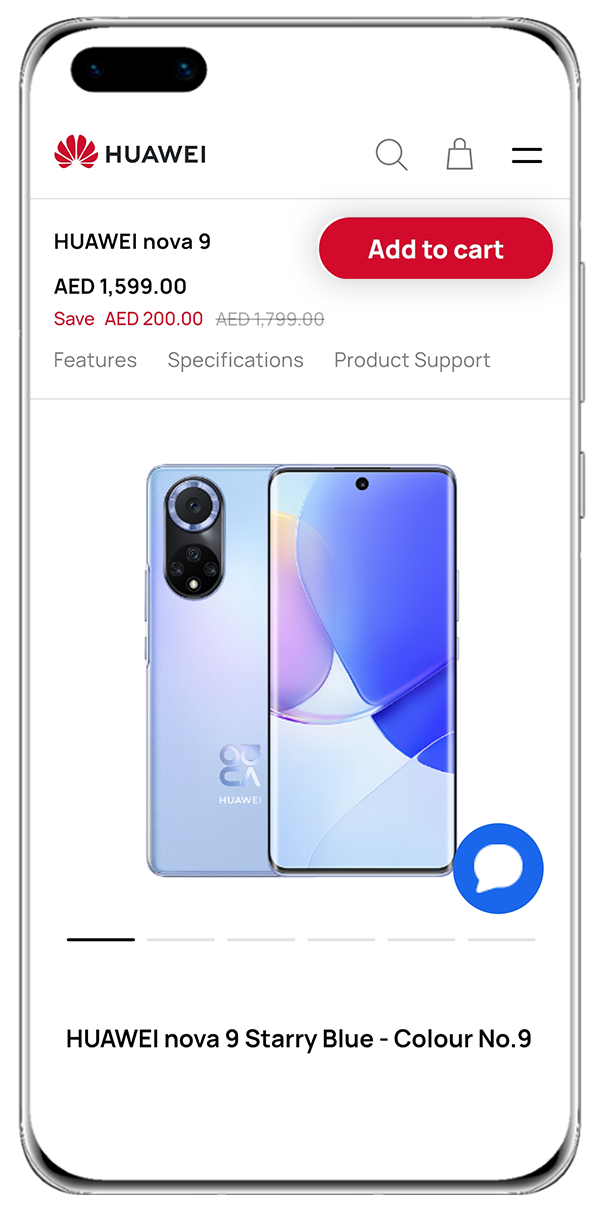A digital promotional image showcasing a cell phone is depicted in this detailed screenshot. The image features a vertically oriented phone with a sleek silver frame. The top left corner of the phone's frame houses multiple camera apertures, while the remainder of the front is occupied by the screen displaying a product listing webpage.

In the top left corner of the phone's display, the brand name "HUAWEI" is prominently written in black, accompanied by a red peacock-style logo to its left. The right side of the top header features a magnifying glass icon (likely for search), a lock symbol, and a two-bar hamburger menu, suggesting navigational options.

Below this header, there's a section providing detailed information about the phone, including its price, clickable buttons for features, specifications, and product support. A prominent red button labeled "Add to Cart" in white text is also present, encouraging viewers to make a purchase.

The central part of the screen is dominated by a large image displaying both the front and back of the phone. The front side showcases a vibrant purple and dark blue screen saver, while the back is adorned with a light sky teal color. 

Towards the bottom right, a blue circle with a chat icon in white indicates customer support or live chat options. At the very bottom of the display, the phone is identified as the "HUAWEI Nova 9, Starry Blue - Color Number 9," completing this comprehensive promotional layout.